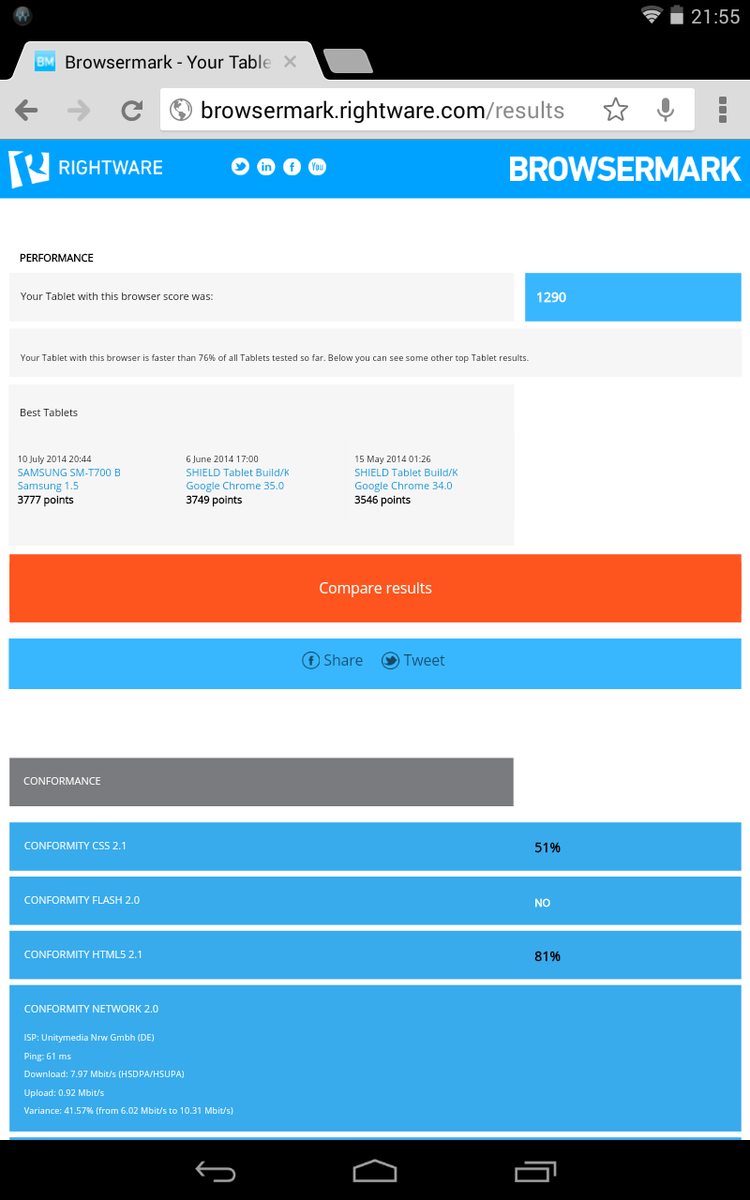This image is a cellphone screenshot featuring a web browser interface. At the top and bottom of the image are black rectangular borders. At the very top, there's a small, partially slanted rectangular box extending into the black border, containing the text "browser mark - your table."

Below this top label, there's a search bar displaying the URL "browser.mark.rightware.com/results." Below the search bar is a prominent blue rectangle. On the left side of this rectangle, there is the text "rightware" next to a logo, which features a white box with an incomplete capital "P" in blue. On the right side of the blue rectangle, in capitalized white text, is the label "browser mark."

Beneath this blue rectangle, there are several gray boxes with text inside them. Under these gray boxes, there's a horizontal orange rectangle spanning the width of the screen, followed by another blue rectangle beneath it.

Toward the bottom of the screen, after some white space, there's a gray rectangle starting on the left side of the screen and extending about two-thirds of the way across. Below this gray rectangle are four smaller blue rectangles lined up horizontally. Each blue rectangle contains very small white text on the left, and they are separated by bright white horizontal lines.